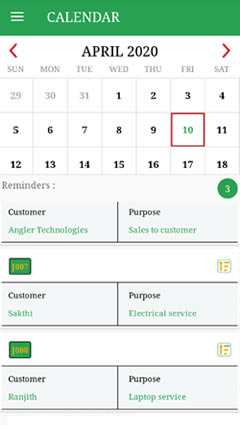The image is a screenshot of a digital calendar app displayed on a mobile device. At the top of the screenshot, there's a green bar with the word "Calendar" written in a white font. The calendar is set to April 2020, and the selected date is the 10th, which falls on a Friday.

Below the calendar grid, there is a list of tasks or appointments categorized by customer names. There are three customers listed: Angler Technologies, Sakia, and Renjia. Each customer has a specified purpose outlined beside their name. For Angler Technologies, the purpose is "Sales to Customers." For Sakia, it is "Electrical Service." For Renjia, the purpose is "Laptop Service."

The layout and functionality of the app suggest it is used as an agenda or task planner, helping the user organize and track various appointments and services associated with different clients.